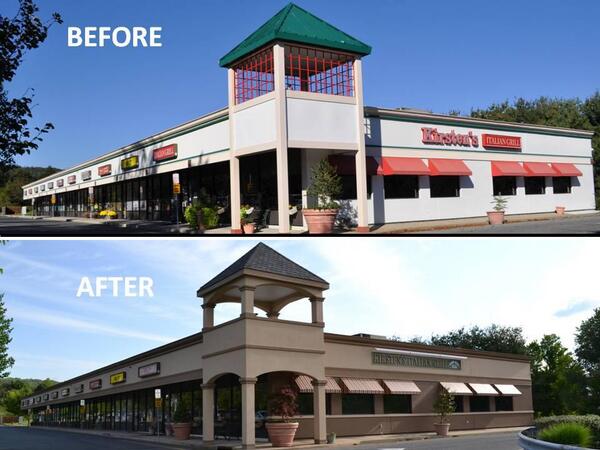This before-and-after image showcases the transformation of a shopping center. In the "before" photo, the shopping center is predominantly white, with a distinctive central gazebo-like structure featuring a green, two-tiered roof and red mesh-like netting beneath it. The right side of the image highlights Kirsten's Grill, while the left includes several unreadable storefront signs. The window dressings and trim are light red. The surrounding area includes visible trees under a bright blue sky.

The "after" photo reveals a significant upgrade. The once-green peak of the gazebo area has been retiled with a black roof, and the red mesh netting has been removed. The entire building has been repainted to a modern, darker cream with brown accents, replacing the previous white and cream colors. The window dressings have been updated to match the new beige color scheme, and there are more prominent, elegant pillars. Some storefront signs have also been updated, contributing to the refreshed, contemporary appearance of the shopping center.